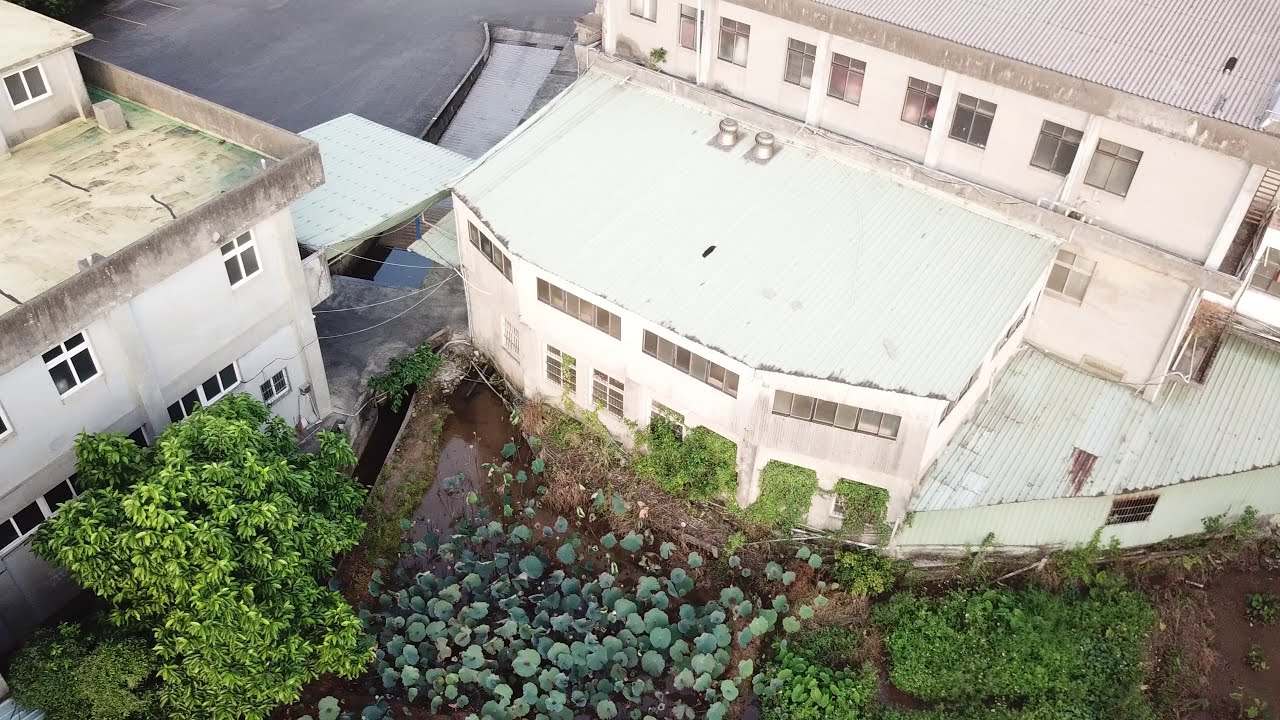This photograph features a top-down, aerial perspective of two industrial, unoccupied buildings. The building on the left side of the frame is a two-story cement structure with numerous white-framed windows. Its rooftop, characterized by a cement balcony area, is partly covered in green grime and hosts a small additional structure with gray walls. The building on the right, also made of cement, features a ribbed metal roof and multiple windows, some of which have trees or shrubs growing out of them, giving a sense of abandonment. In the foreground, there's brown, muddy dirt with a variety of trees and large green-leafed plants, resembling a garden or natural overgrowth. A cement parking lot or pad is visible in the distance, adding to the desolate industrial atmosphere. No people or text are present in the image.